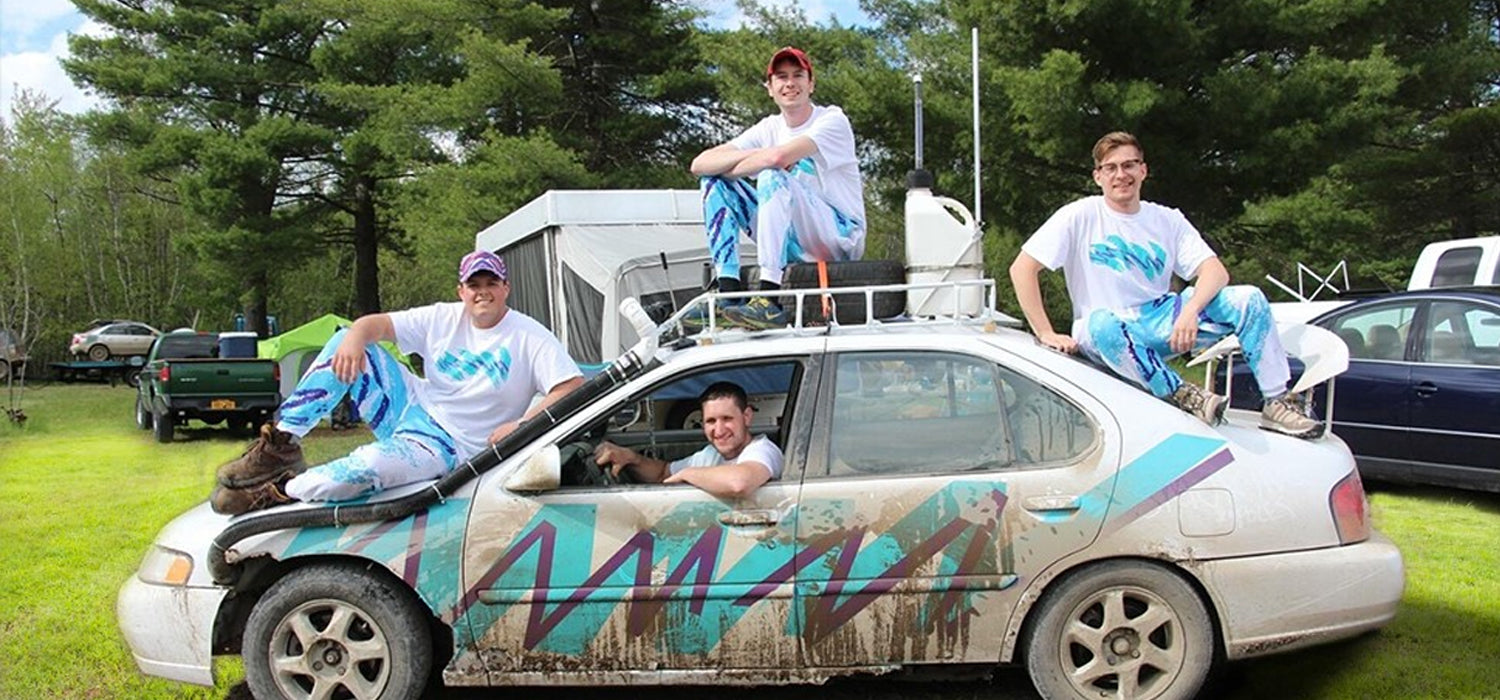This color photograph captures a scene in a grassy field, possibly at a campground or festival, with a distinctively marked, old, and dirty white car that features prominent purple and turquoise zigzag stripes along its sides. Surrounding the car are four young white men, all seemingly in their early 20s, with three standing beside or sitting on the car, and one in the driver’s seat. All the men are looking proudly at the camera and wearing matching white t-shirts and pants adorned with the same zigzag pattern as the car.

The driver, who is smiling, has one hand on the steering wheel and the other arm propped up against the door. The car’s peculiar appearance includes scuff marks, mud splatters, and general wear. There’s a jug or gas can positioned near the man sitting on the back part of the car, who wears glasses and has his jeans featuring the zigzag pattern. Another man sits on the hood of the car, also in a white shirt and zigzag-patterned jeans, while the third man, perched on something atop the car, wears a ball cap.

In the background, various vehicles are visible, including a blue car, a pickup truck, a trailer, and the top of a tent, with a heavily wooded area nestled further back. This lively and cohesive scene suggests a shared event, conveying camaraderie and a potential theme among the group present.